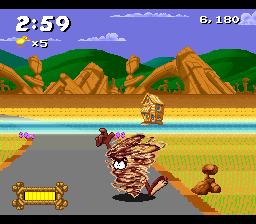This is a cover screenshot from an older video game, evident from its pixelated graphics. The scene features a detailed and vibrant landscape. A tranquil water body, represented by a blue line across the middle of the image, dominates the foreground. Centrally located within this water body is a charming, rustic two-story wooden building, adding a quaint touch to the scenery.

In the background, rocky structures emerge, providing a rugged contrast to the surrounding tall, green hills that frame the image. The sky overhead is a bright blue, adorned with a smattering of fluffy white clouds, enhancing the overall picturesque quality of the setting.

Prominently featured in the center is the iconic Tasmanian Devil from the Looney Tunes cartoon series. He is depicted in his signature style as a chaotic, whirling brown tornado. From this whirlwind, his arm juts out from the top, and his two white eyes peer from the center whirlwind, while his left foot sticks out, amplifying his dynamic and frenetic energy.

Additional game elements are visible: at the top left, the numbers "2:59" are displayed, possibly indicating the time remaining. Near this, a small, cartoonish yellow bird appears with the notation "x5," suggesting a multiplier or quantity. In the top right corner, the current score is prominently displayed, reading "6180."